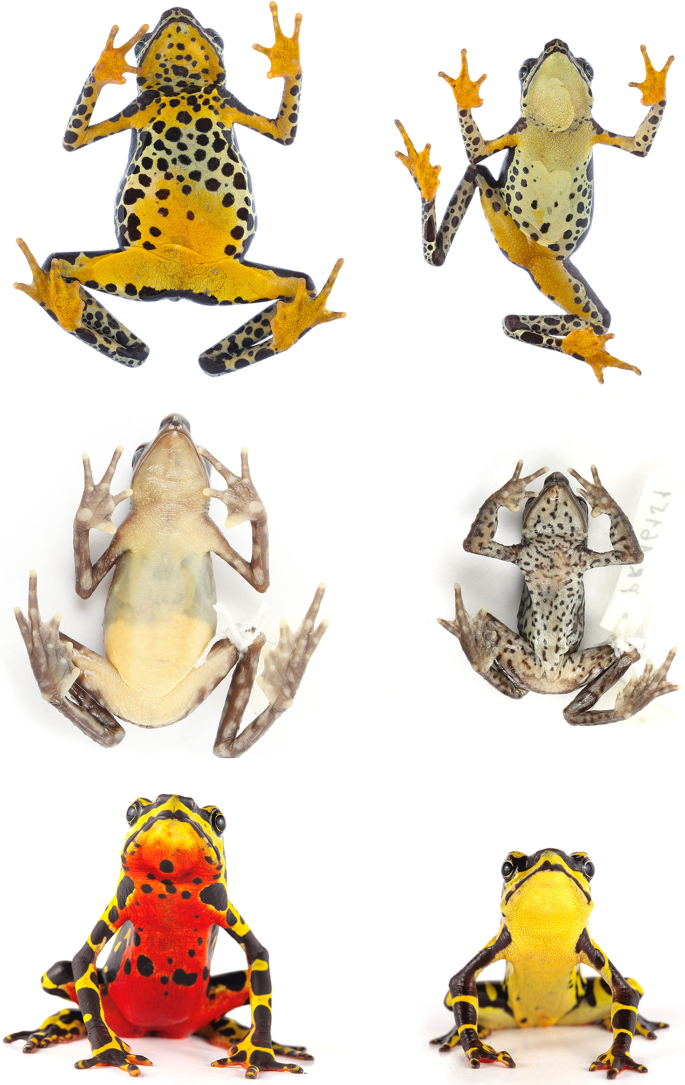The image showcases six different frogs, each uniquely colored and patterned, arranged against a white and black background. Positioned in a grid format with two frogs across and three down, the top two frogs resemble leopard frogs with black spots on their yellow bodies, although the one on the left has more prominent markings. The middle left frog has an almost completely white underbelly with some gray and brown on its legs, while the center right frog is smaller and grayish with black spots covering its entire body and legs. The bottom row features two frogs in a more frontal view, allowing their eyes to be visible. The lower left frog has an orange underbelly with black spots and little orange feet, and the frog to its right has a yellow body with black legs and two visible eyes. The diverse and vivid coloration, including a red frog with spots and one with a clear yellow underbelly, raises the question of whether these are artistic depictions rather than photographs of real frogs.